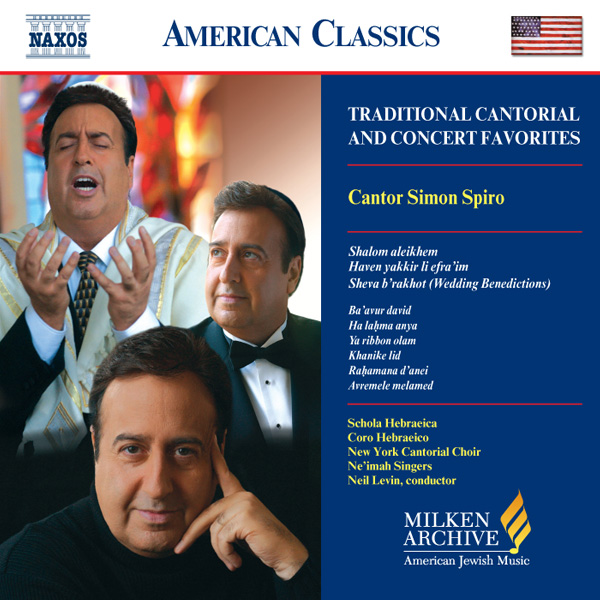The image is an advertisement for concerts or possibly the cover of a CD album. Dominating the top section, the title "American Classics" is displayed prominently in blue, with an American flag positioned to its right. Below this, to the left, there is a composite photograph that features three images of the renowned Cantor Simon Spiro in different poses and outfits. 

The topmost photograph captures Simon Spiro singing passionately with his arms outstretched and his eyes closed, a backdrop of stained glass adding a solemn touch. The middle image shows him in a tuxedo with a black bow tie, gazing upward thoughtfully. The bottom photograph presents Spiro in a black turtleneck, his hand resting on the side of his face with his index finger touching his temple, looking directly at the camera with a gentle smile. 

Adjacent to these images, running vertically on the right side, is a blue bar containing the text "Traditional Cantorial and Concert Favorites" in white, followed by the name "Cantor Simon Spiro" in yellow. Below this, the text lists various traditional songs and choirs involved, including: "Shalom Aleichem, Havan Yikir Le Efraim, Sheva Barakot - Wedding Benedictions, Baavar David, Alakma Anya, Yaribon Olam Kanikeleid, Rahamana Dansi, Avevemele Melamed." The choirs mentioned are "Skola Ebreika Koro Abratziko, New York Cantorial Choir, and Naima Singers" with Neil Levin as the conductor. The bottom of this section features the logo for the Milken Archive of American Jewish Music, accompanied by the description "Milken Archive of American Jewish Music" at the bottom.